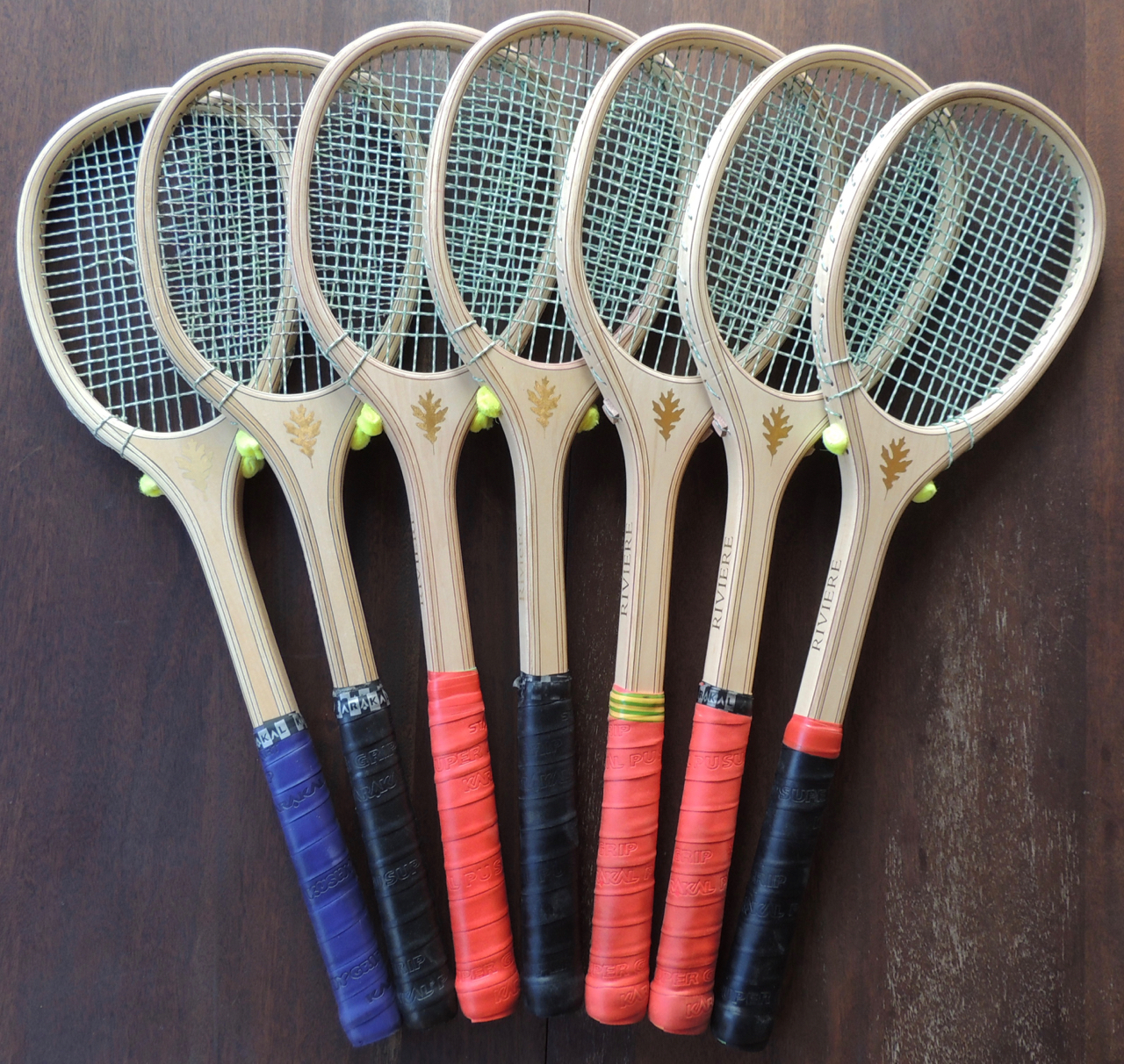This image features a set of seven wooden-framed rackets, likely tennis or racquetball, arranged in a fanned-out, overlapping manner on a dark brown wood grain surface. The rackets share a uniform shape with rounded tops, unfinished wood appearance, and a leaf emblem situated below the netted area, which consists of white and black crisscrossing lines. The handles are wrapped in grips of varying colors: the first is light blue, followed by black, bright red, black again, another bright red, a slightly darker red, and finishing with black. The surface beneath shows green marks and a mix of smooth and rougher textures, with some wear visible as whitish-gray areas. Some rackets bear the name "Revere," indicating the manufacturer.